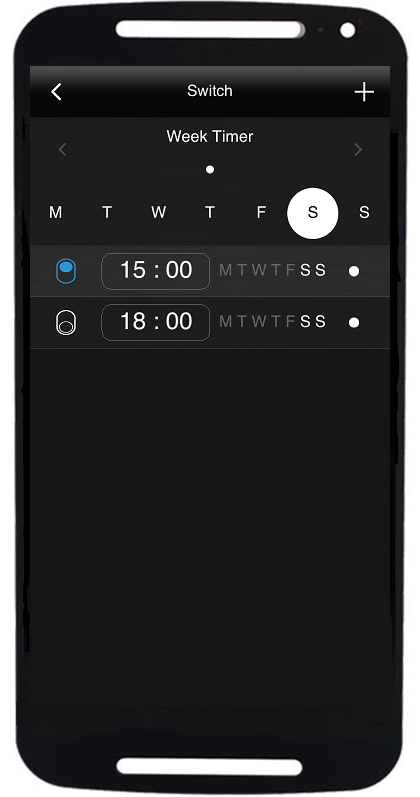The illustration depicts a black cell phone displaying the alarm app interface. The screen is free from any indicators such as time, date, carrier, Wi-Fi, service signal, or battery percentage, highlighting that this is a graphical representation, rather than a real phone. 

At the very top, a black bar spans the screen containing the word "Switch" with a left-facing arrow for navigation. On the opposite side of this bar, there is a plus symbol for adding new alarms. Below this bar, the screen features a "Week Timer" section with left and right arrows, allowing the user to switch between weeks. Positioned centrally is a white dot.

The days of the week are represented by the letters "MTWTFSS," with Saturday highlighted by a white circle. 

At the bottom part of the interface, there are two alarms set: one for 15:00 (3:00 PM) and another for 18:00 (6:00 PM) displayed in a 24-hour format. The first alarm, set for 15:00, is turned on, indicated by a blue toggle switch in the upward position. The second alarm, set for 18:00, is turned off, with its toggle switch in the downward position. The active alarm applies to both Saturday and Sunday.